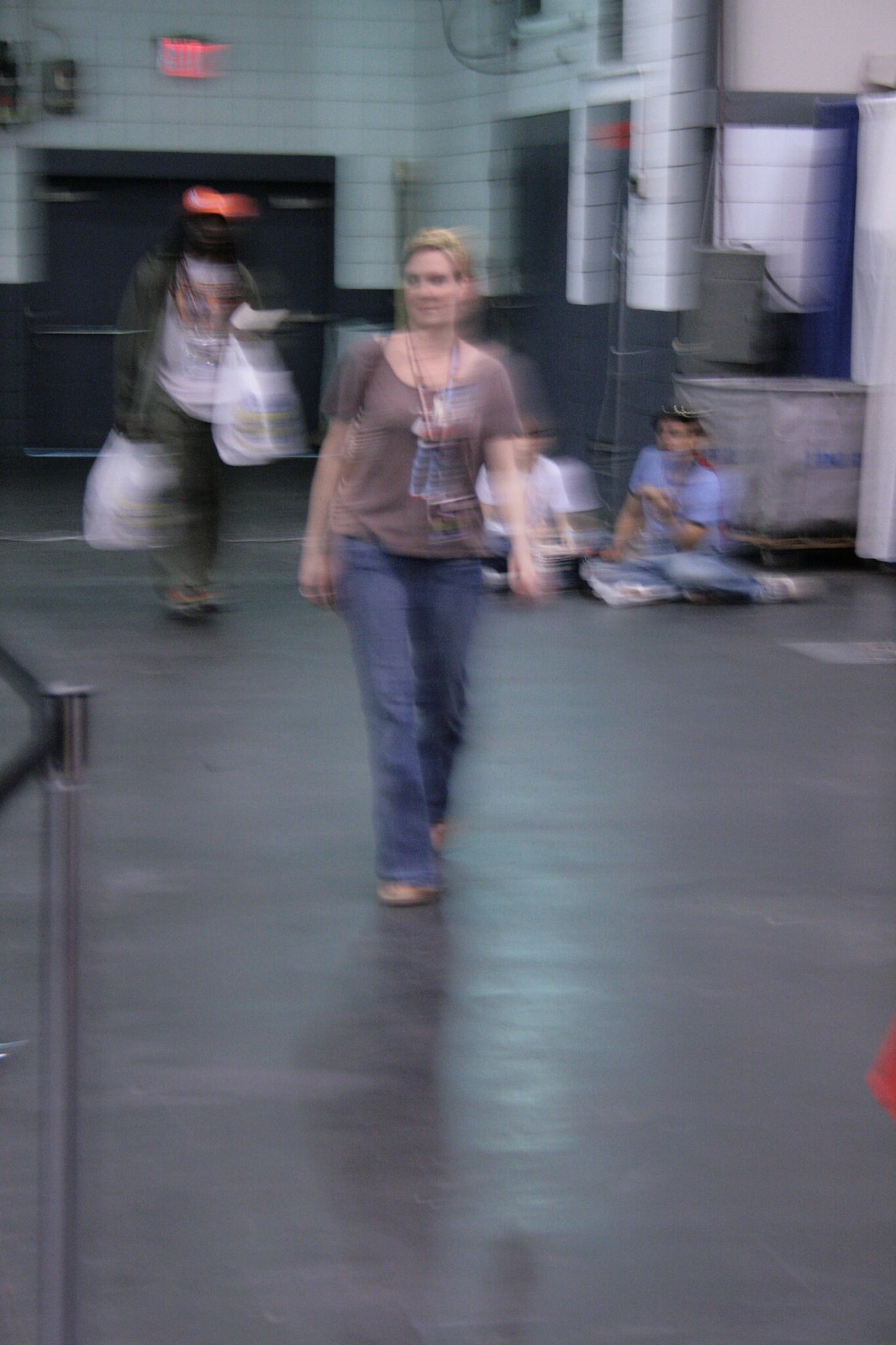The image is a vertical, blurred photograph capturing a scene inside what appears to be a warehouse or convention center with a white brick wall and a gray cement floor. The focal point of the image is a blonde woman with fair skin, wearing flared blue jeans, a brown top, and a lanyard. She appears to be walking towards the camera with a handbag on her right shoulder. Behind her to the right, two people are sitting on the floor; one is wearing a blue outfit consisting of jeans and a light blue t-shirt, while the other wears light blue jeans and a white t-shirt. Further in the background, there is a black man with long hair, wearing green slacks, a graphic white t-shirt, and a green zip-up jacket. He is holding two white bags and wearing a red cap. The setting includes a gray pushcart, a red exit sign, black double emergency doors, and various pieces of wiring on the white brick wall. There is a general haze pervading the image, making facial expressions and finer details indistinguishable.